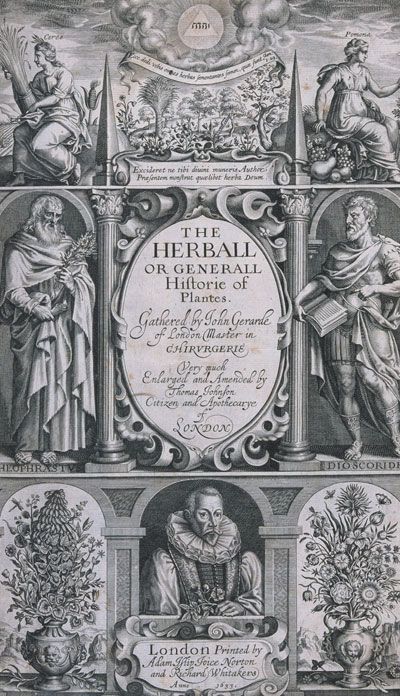This image appears to be a detailed black-and-white engraving of an old book cover, possibly dating back to Roman or Elizabethan times. The cover is ornately divided into three sections, each featuring distinct illustrations and text. The top section showcases a woman looking left and holding a stalk of wheat, flanked by Latin script on banners. The central section, dominated by an oval crest, contains the title "The Herbal or General History of Plants, gathered by John Gerard of London, Master in Chyrurgry," further elaborated with "very much enlarged and amended by Thomas Johnson, Citizen and Apothecary of London." This section also depicts a man with a beard on the left, holding a leaf and perhaps a candle, while another man on the right carries a book and gestures towards it. The bottom section features a central figure with a large Elizabethan collar, possibly indicative of Shakespearean times, surrounded by potted flowers. The text at the bottom reads "London, printed by Adam Joyce Norton and Richard Whitakers," though it is small and somewhat difficult to decipher. Overall, the cover art showcases figures in robes, ancient styling elements, and decorative plant illustrations, weaving together themes of history, botany, and classical literature.